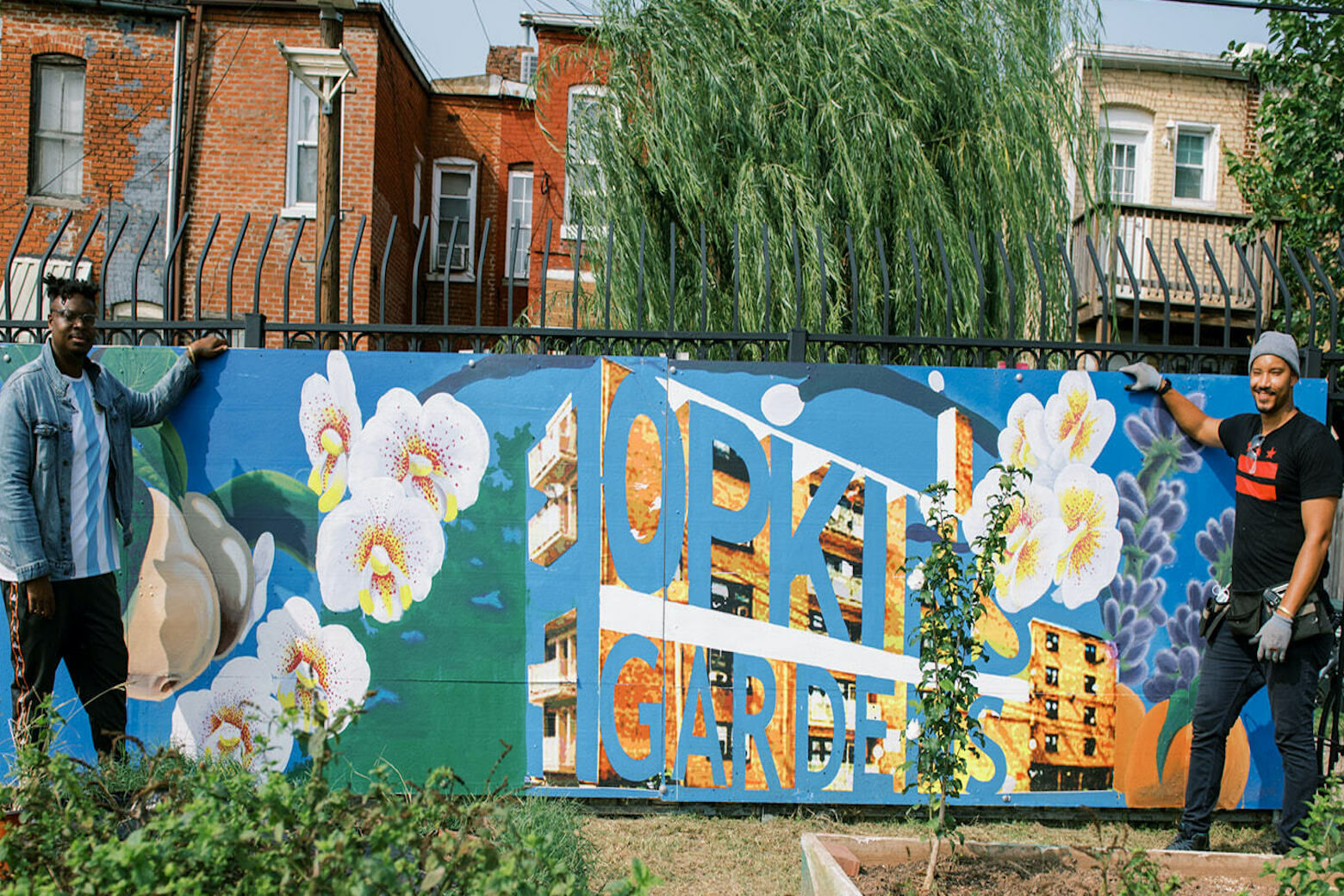This vibrant color photograph captures a lively city scene bathed in sunlight. In the background, a series of row houses or apartment buildings, constructed from red and beige bricks, stand closely together, reflecting the architectural style of the late 19th to early 20th century with their white window panes. In the foreground, there is a thriving urban garden featuring various flower beds and green vegetation. Dominating this area is a large mural attached to a black wrought iron fence. The mural is brightly painted with illustrations of flowers and vegetation and prominently displays the words "Hopkins Gardens" in large blue text. Positioned beside the mural are two smiling black gentlemen, likely in their 20s or early 30s. The exact nature of their involvement with the mural—whether as its creators or caretakers of the garden below—remains unclear, but they stand proudly flanking the colorful artwork, adding a personal and human element to the community-centric scene.